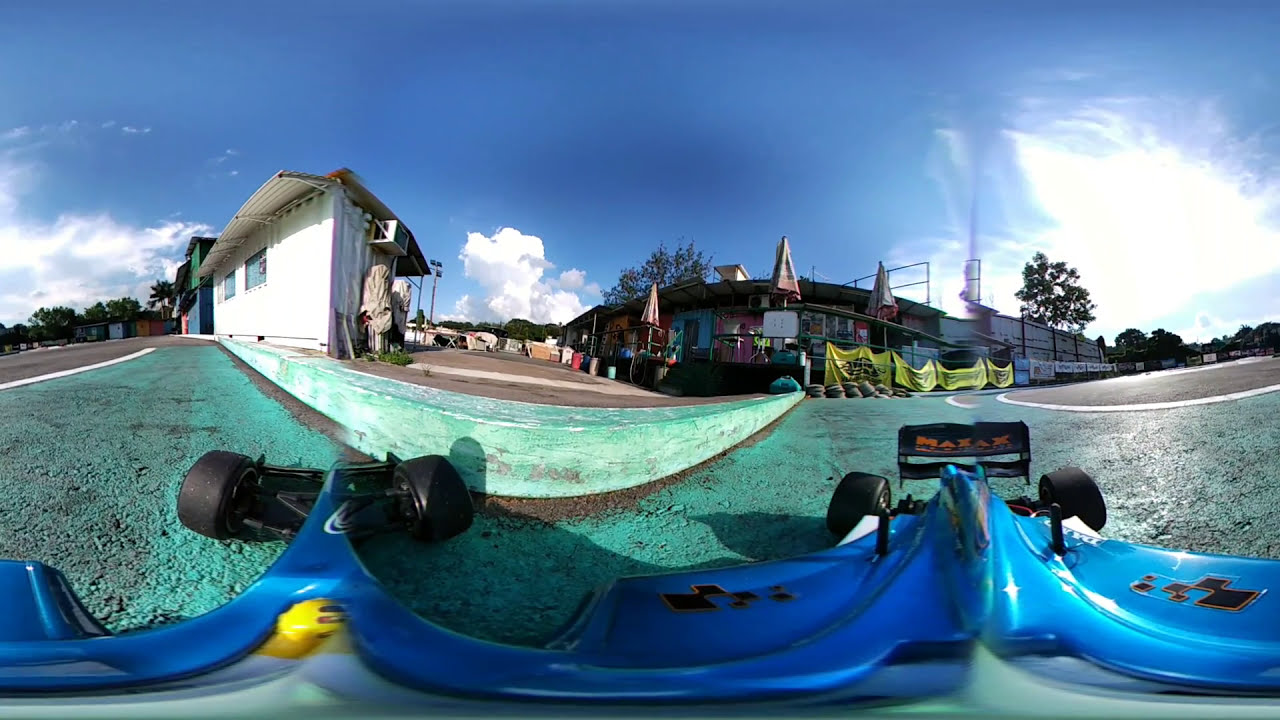This photograph, captured from inside a blue, F1-styled go-kart, appears distorted due to a fisheye filter, giving it a 360-degree effect that shows both the front and back of the go-kart. The black tires of the go-kart contrast sharply with the light blue-painted track it is driving on. To the right of the go-kart, the track transitions to a grey color, and scattered tires can be seen lying on the road. Surrounding the track, a variety of buildings and houses are visible, including structures that look like shacks with white walls and blue windows. One of the central buildings features a mix of blue, purple, and red colors, with folded umbrellas on the top and a thin fence lining it. Additionally, the sky above is a vivid blue with white clouds, trees, and the sun visible on the right-hand side. The go-kart's rear fender bears the word "MAXAX," and along the buildings, banners and rails are noticeable, adding to the scene's detailed urban backdrop.